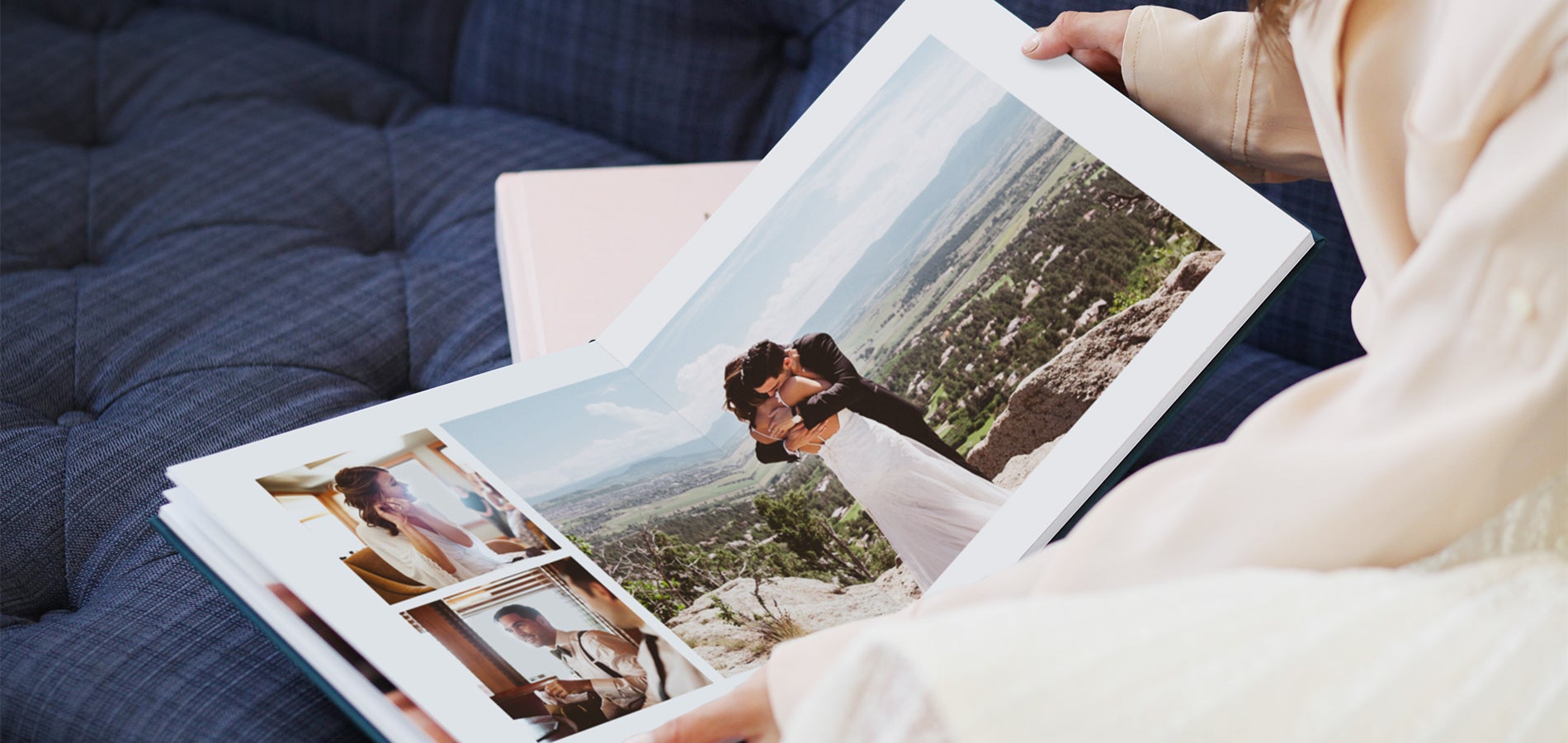In the image, a person, possibly a female, sits on a pleated navy blue couch adorned with button dimples and examines a wedding photo album. She is dressed in all-white clothing, possibly a white dress shirt or khaki-colored loungewear. The photo album is fully open, and she holds it with both hands while looking intently at the pictures. The central photograph depicts a man and a woman standing on a rocky cliff with large gray rocks, surrounded by lush greenery and numerous mountains in the background. The couple is hugging; the woman, dressed in a long white dress, is embraced from behind by the man in an all-black suit. Both appear to be Caucasian. Other images in the album include moments of the woman getting ready for the wedding and the man holding a cocktail glass without his suit coat. The scene portrayed seems reminiscent of a picturesque landscape, possibly akin to New Mexico.